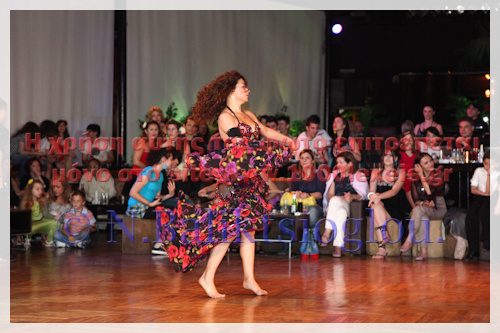The photograph captures a woman deeply engrossed in a dance performance on a shiny, wooden floor, barefoot. She has curly, dark brown hair that falls just below her shoulders and a light-colored skin. She wears a striking, sleeveless floral dress that is predominantly black with vibrant red accents, featuring a halter top. Her hands are raised gracefully. The backdrop includes white curtains and an audience composed of mostly adults seated on chairs, with some children sitting on the floor. While many spectators are focused on her performance, some are distracted, engaging in conversation or looking elsewhere. Additionally, part of the woman is partially obscured by text in a foreign language on the image. A single white light illuminates the scene from the left side, adding depth to the composition.